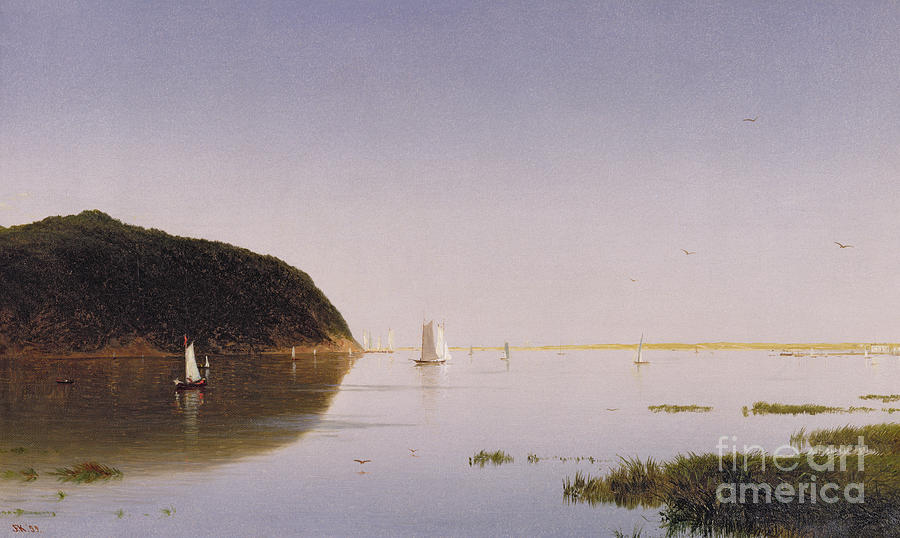This is an outdoor photograph taken during the daytime, depicting a tranquil lagoon or harbor. The foreground features a body of light blue-gray water, densely populated with numerous sailboats, most of which have white sails. Some boats are in the shallow, calm waters near the jetty area. At the bottom right, a small patch of grass extends into the water, with seaweed visible near the surface. 

To the left, a prominent, large rock formation or cliff is visible, partially covered with forested growth including trees and bushes, and it slopes down to the water. The horizon showcases a muddy yellowish land, possibly due to natural terrain or lighting effects. 

The expansive sky above dominates most of the image, scattered with birds, including three seagulls flying towards the right. Furthermore, the photograph contains a watermark in the lower right corner that reads "Fine Art America." No shadows are visible, and the sun isn’t directly seen in the frame, emphasizing a serene and even lighting across the scene.